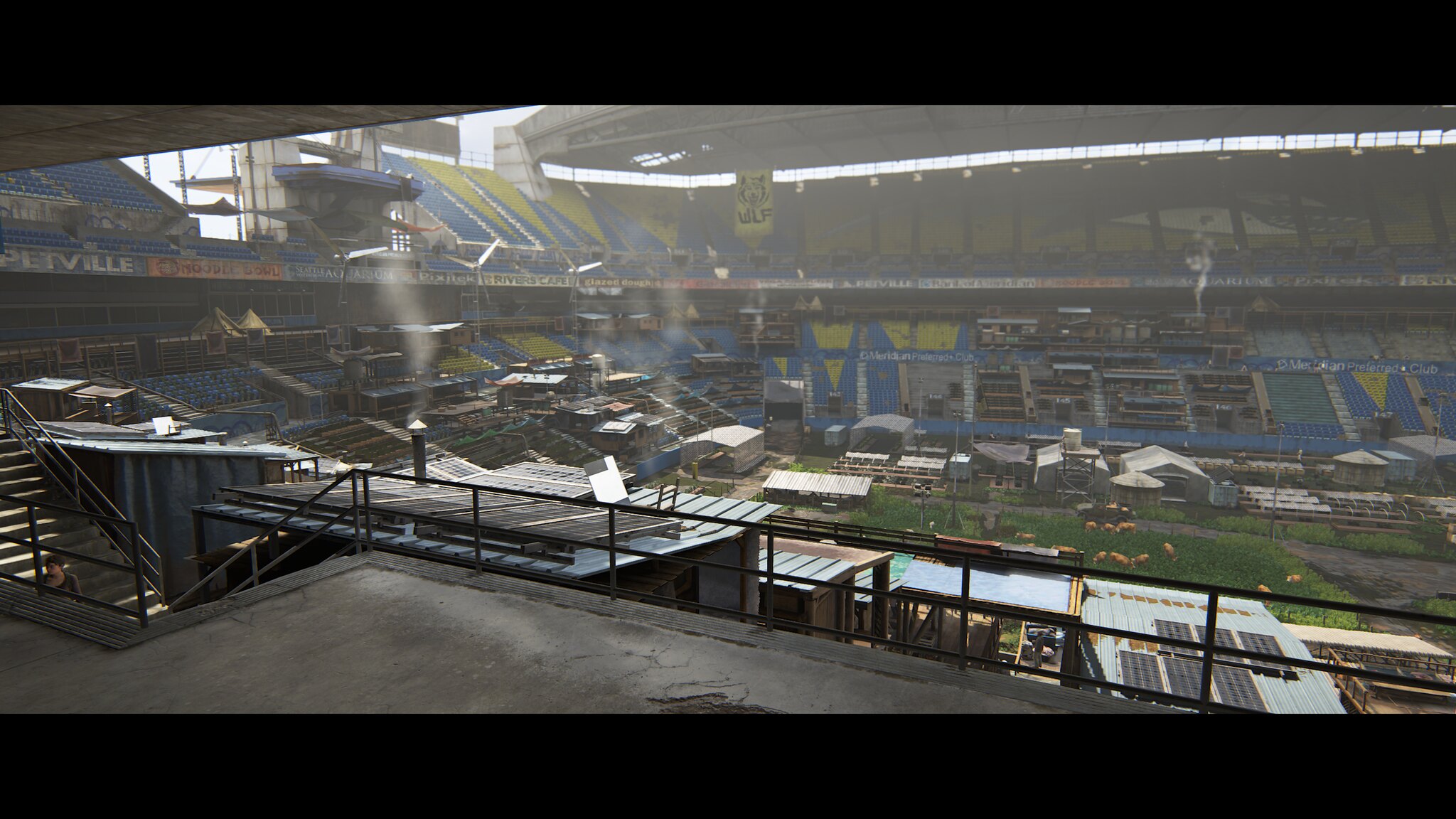The image depicts the inside of an abandoned, two-level stadium, characterized by blue and yellow seats forming an upside-down yellow triangle pattern from the top to the bottom rows. The photograph is taken from the mid-level seats, providing a sweeping view across the field. The stadium's lower-left seating area appears damaged or disarranged. The lush green field at the center is segmented by asphalt paths, suggesting the space is no longer used for traditional sports. Scattered across the field are numerous small white tents and structures resembling picnic tables or temporary huts and barns, which imply usage for a livestock show or a farmers' market. In the background, there's a large open glass structure with a blue roof, possibly housing an announcer's booth. A smokestack emitting smoke rises from the middle of the field, and the entire scene appears to be set in a post-apocalyptic context, reminiscent of a setting from 'The Last of Us 2.' The stadium shows signs of decay and repurposing, with scaffolding, sponsorship signs that are difficult to read due to blurriness, and a lone visible person navigating the tan concrete stairs with metal railings.